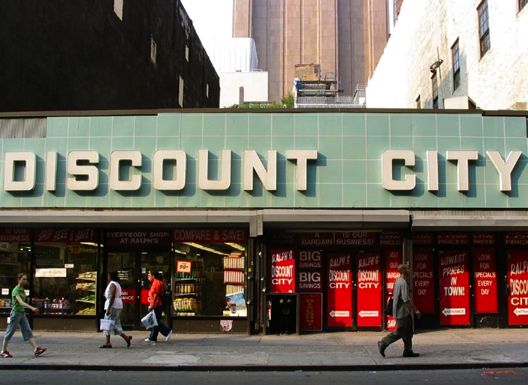This photograph captures an aged storefront named Discount City, likely taken around 20 years ago, given the quality of the image. The store's prominent sign, "Discount City," is displayed in white lettering on a backdrop of light blue tiles, some of which are missing, adding a touch of wear to the scene. Below the sign, a series of glass windows adorned with various red and white advertisements catch the eye, each promoting enticing offers like "Lowest Prices in Town," "Look for Specials Every Day," "Everybody Saves," and "Compare and Save." These banners often feature white arrows guiding the viewers' attention around the store. Displayed within the windows, assorted products are visible, though specific items are indistinguishable.

In front of the store, a broad sidewalk bustles with activity. Several people are depicted walking in various directions. Notably, one person dressed in a grey t-shirt, black trousers, and black shoes moves to the right, while others, including two wearing white shirts and blue jeans, traverse the pathway. One individual in green and blue shorts with red shoes strides to the right, contributing to the lively atmosphere.

Behind Discount City, the urban environment extends with additional buildings in the background—a black one with white windows to the top left and a white building with glass windows to the top right. Moreover, some greenery can be spotted on these structures, further enhancing the city's textured layers.